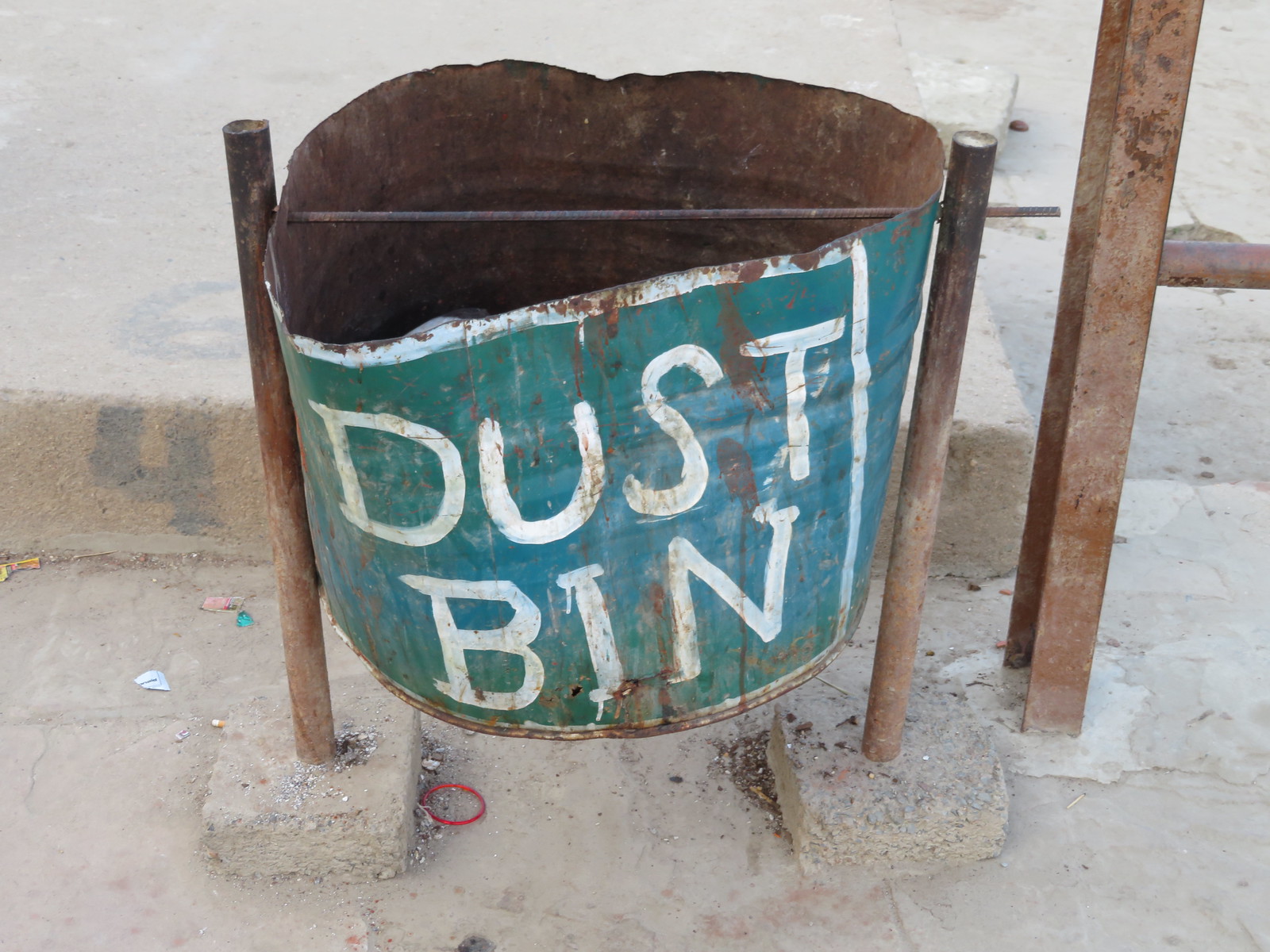This photo depicts an old, vintage dustbin positioned on the side of a street. The central focus of the image is a circular metal dustbin painted in a greenish-blue color, with the word "dustbin" hand-painted in white letters within a bordered square. The bin is rusted both inside and out, with visible holes drilled through its sides, allowing it to hang from a small metal rod. This rod is suspended between two larger, rusting vertical poles, which rise from square concrete bases embedded in the pavement.

To the right of the dustbin, there is a partially visible angle arm and a bar, hinting at other structures just outside the frame. On the ground beneath the dustbin, several small objects are scattered, including a red rubber band or hair tie, a blue marble, fragments of yellow and blue paper, and a penny. The setting appears to be outdoors, in a public area, possibly in the middle of the day, situated on a stone surface with a curb visible in the top left of the image. 

The color palette includes tan, blue, white, green, red, gray, and brown, enhancing the scene's nostalgic and slightly neglected atmosphere.